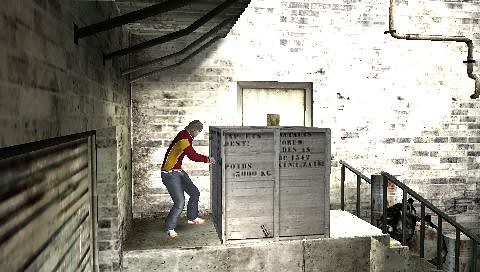The image appears to be a screen capture from a video game. The scene is set against the exterior wall of a warehouse near a shipping bay or loading dock. The warehouse wall is constructed from a mix of gray and white bricks, giving it a stark, monochromatic appearance. 

At the bottom center of the image, there is a cement platform reached by three cement steps on the right side, which are equipped with black metal railings on either side. Positioned centrally in front of a door area behind it is a large shipping container marked with black lettering.

To the left of this container stands a man dressed in a red and yellow striped shirt, gray pants, and white sneakers. He appears to be attempting to break into or open the container from its left side. To the left of the man is another section of the building's wall, also made of gray and white bricks, featuring a grayish awning overhead.